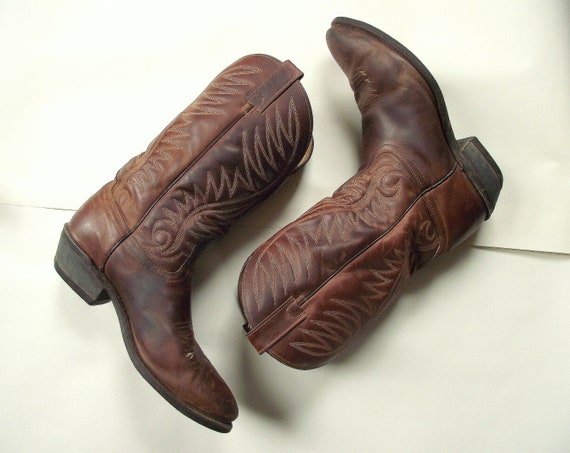This is an overhead photograph of a pair of well-worn, yet well-cared-for, men's brown leather cowboy boots. The boots are placed in a yin-yang or 69 position with the shins parallel to each other and the feet pointing in opposite directions. The gradient shading on the boots transitions from a dark brown at the toes to a lighter shade towards the shafts. Intricate white stitching, resembling flame patterns, adorns the leather. The background of the image is a neutral tan, and it appears there may be a white paper overlay running vertically through the center, enhancing the visual contrast. These seasoned boots are artfully displayed as both a testament to their rugged use and the care they've received.